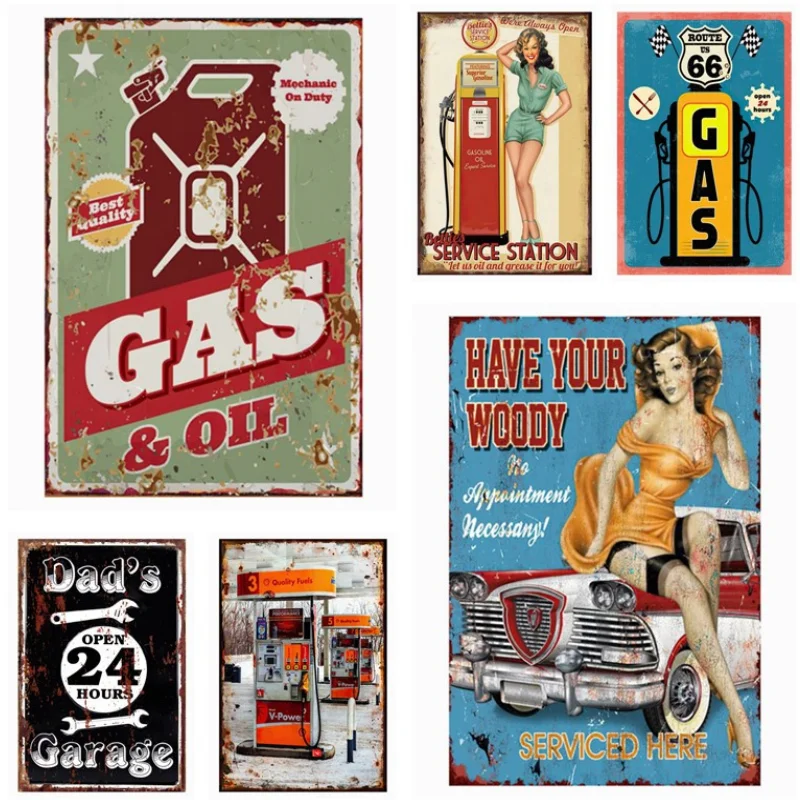This illustration showcases a collection of six vintage advertisements from the 1940s or 50s, most of which appear on rusted metal signs. The top-left features a light green sign with a distressed red gas can labeled "Best Quality," "Mechanic on Duty," and prominently "Gas & Oil," with the words "Gas" in white on a red parallelogram background. Adjacent to this is Betty's Service Station's poster, sporting a white and tan background. A pin-up style lady in green poses beside a red and yellow gas pump, promoting, "Let us oil and grease it for you." Next, a blue-themed sign showcases a yellow gas pump with the Route 66 logo and checkered flags. 

The bottom row highlights a larger, saucier advertisement featuring a pin-up model in a yellow dress seated on a red and white '57 Chevy, captioned boldly in red and white: "Have your Woody serviced here. No appointment necessary." Directly to her left, a modern Sunoco or Shell gas pump is depicted, suggesting "Quality Fuels," although it appears more contemporary with a snowy backdrop. Finally, the far left image has a black background with faded text reading "Dad's Garage, Open 24 Hours," accompanied by wrenches, evoking a timeless service appeal. Each sign reflects the era's charming blend of art, advertising, and automotive culture.